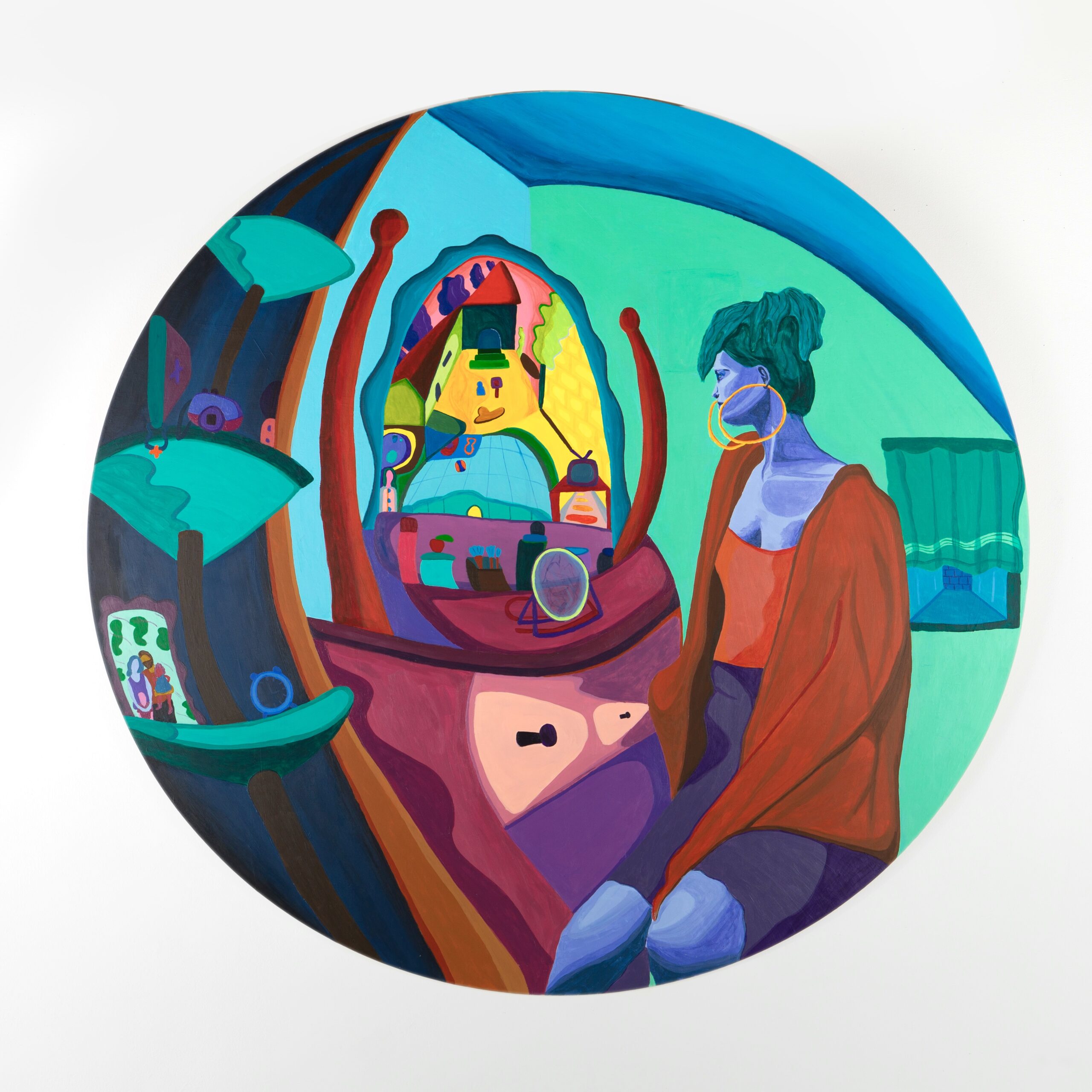The image depicts a surreal, abstract painting featuring a woman with bluish-purple skin and teal green hair. She is seated within a round composition against a grayish-white background. The woman wears a red jacket over a red top and a navy blue skirt, accentuated by large gold hoop earrings. Positioned in profile, she gazes into a mirror, which intriguingly presents an alternate scene rather than reflecting her visage. This alternate reality within the mirror includes various elements like a lamppost, picture frame, a television or swimming pool, and a curtain that partially reveals the outside world. The setting around her is vibrantly colored with seafoam green and light blue walls, along with a dark blue ceiling, adding to the overall surreal and distorted fisheye effect that makes the environment appear skewed and dreamlike. The dresser in front of the woman, although meant to reflect, instead showcases an eclectic array of colors and shapes, enhancing the whimsical and otherworldly nature of the artwork.